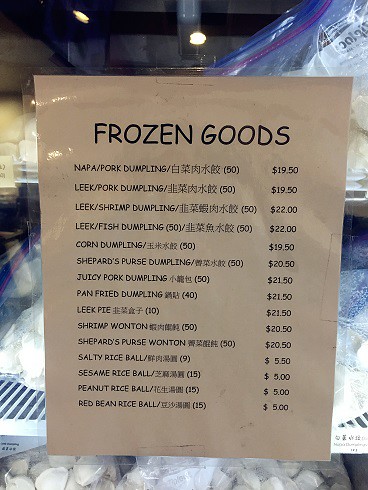Close-up indoor color photograph depicting a piece of white paper taped to a window. The paper is a price list titled "FROZEN GOODS" in black, capitalized print. It features approximately 14 to 15 food items, each described in a left column with both American and Asian characters. The pricing for each item is listed in a right column. The first item on the list is "Napa Pork Dumpling," followed by four or five Asian characters, with a quantity of 50 in parentheses and a price of $19.50. 

In the blurred background, bags of what appear to be small clams are visible, along with the ceiling of a warehouse and one or two lights in the upper left corner. The foreground, including the paper and its text, is in clear focus. This photograph effectively captures a detailed price listing for frozen goods, presumably available for sale at the pictured store or market.